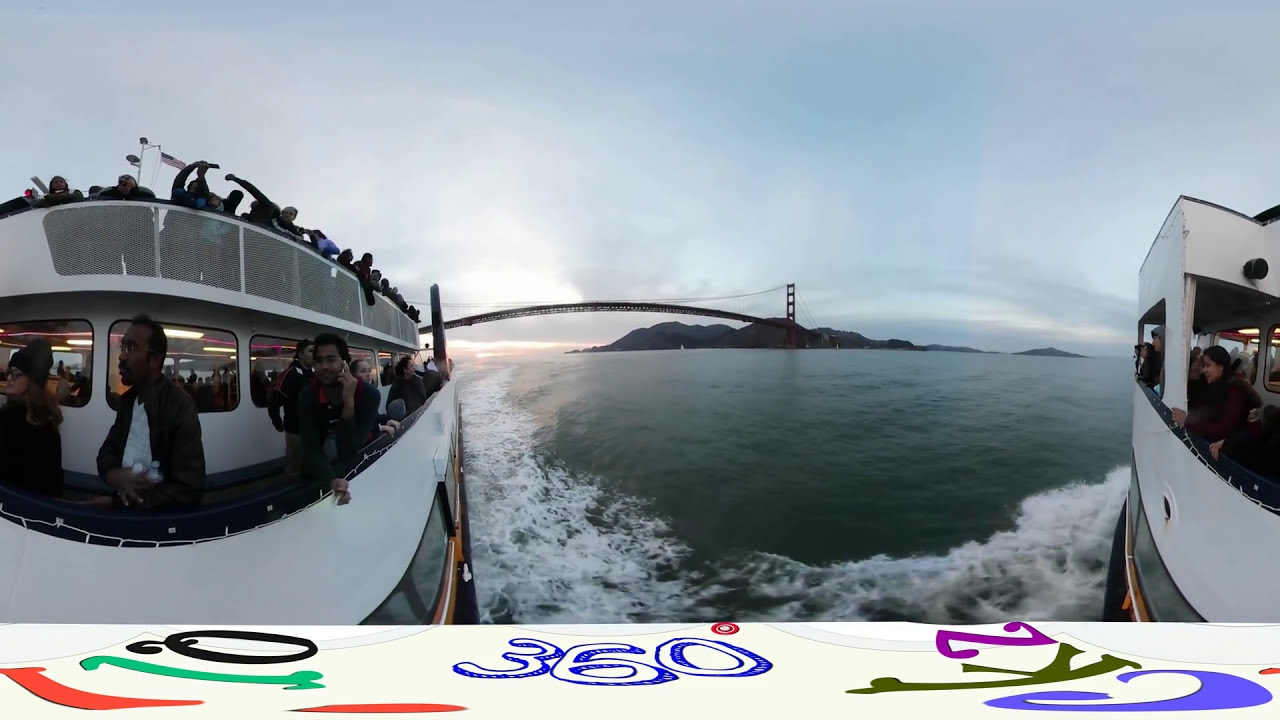This outdoor photo captures two multi-decked boats navigating gray, foamy waters against a backdrop of a hilly landscape, horizon, and a bridge that appears to span from an island to the left. The boat on the left dominates the image, showcasing three decks bustling with people taking photos and observing their surroundings. The boat on the right is partially visible, showing its side with several individuals on the main deck. The San Francisco Bridge is prominently featured, stretching behind the boats. The vibrant color palette includes green, black, red, blue, white, dark green, gray, and orange, with the blue sky enhancing the scene.